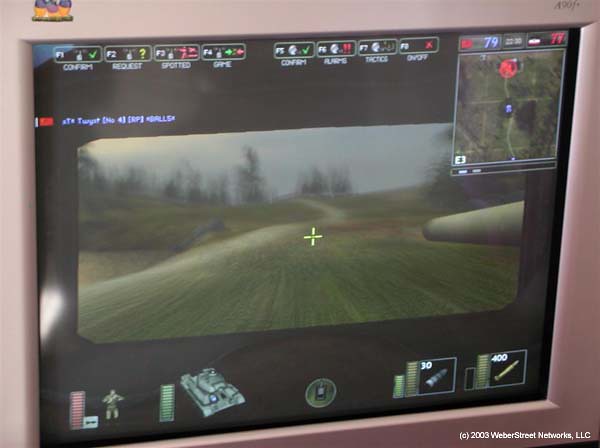The image features a vintage handheld gaming device, distinguished by its pale purplish-pinkish hue. The device's screen, which occupies the central frame, appears relatively small. A copyright inscription at the bottom right corner reads "© 2003 Wiperstreet Networks, LLC." 

Displayed on the screen is a scene from a virtual world game, which seems to be an exploration or war simulation game. The interface is detailed with several gaming elements: a prominent tank, health bars, and a small soldier character, likely controlled or positioned by the player. The ammo count is displayed on the bottom right corner.

At the top of the screen, the word "Stats" is visible, indicating player statistics, while the top right corner shows a map of the game area being explored. The player's view includes a central crosshair for aiming, suggesting a shooting mechanic. The landscape depicted is a grassy plain, with a visible weapon barrel, presumably the player's gun, in a gray hue on the right side of the screen.